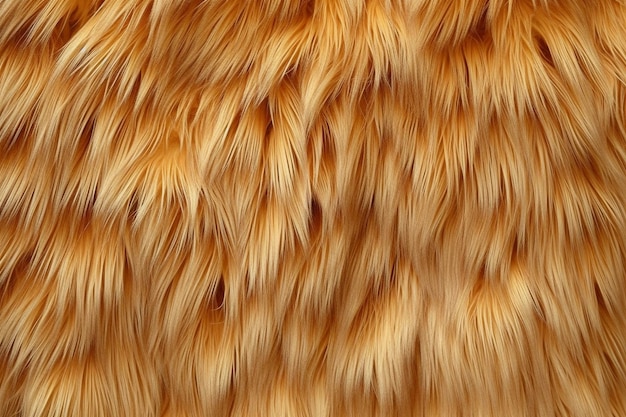This is a detailed photograph showcasing a close-up of wavy hair or fur, which appears to be predominantly golden blonde with varying shades. The hair or fur strands are neatly arranged, cascading from top to bottom within the frame. The image captures the intricate layering, with the roots appearing slightly darker, transitioning through tan mid-lengths and culminating in pale yellow or light orange tips. The texture is uniformly wavy and meticulously maintained, with no visible split ends. The hair or fur is the sole focus, filling the entire rectangular frame, which is wider than it is tall. The precise nature—whether it belongs to a human, an animal, or is perhaps a highly detailed 3D rendering—remains ambiguous, yet the realistic detail suggests natural origins.